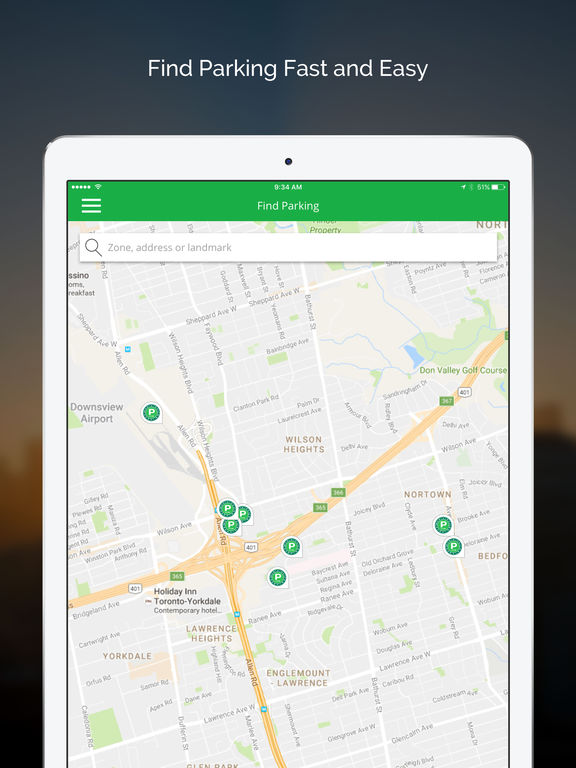The image captures a tablet screen, possibly an iPad, displaying a map application geared towards helping users locate parking spots. The map's focal point is an urban area, likely a section of a city, illustrated with precision. Scattered across various locations on the map are green icons marked with a "P," each symbolizing an available parking spot. These icons offer different parking options for users to choose from. 

At the top of the screen, a green header bearing the white text "Find Parking Fast and Easy" highlights the app's main function. Just below this header, there's a search bar where users can input a zone, address, or landmark to locate specific areas. The map includes several detailed elements, such as street names and notable locations like the Dawn Valley Golf Course and the Downsview Airport.

The user interface is clean and straightforward, characterized by a minimalistic white and green color scheme. Aside from the interactive elements at the top, the UI maintains a simplistic design, emphasizing ease of use.